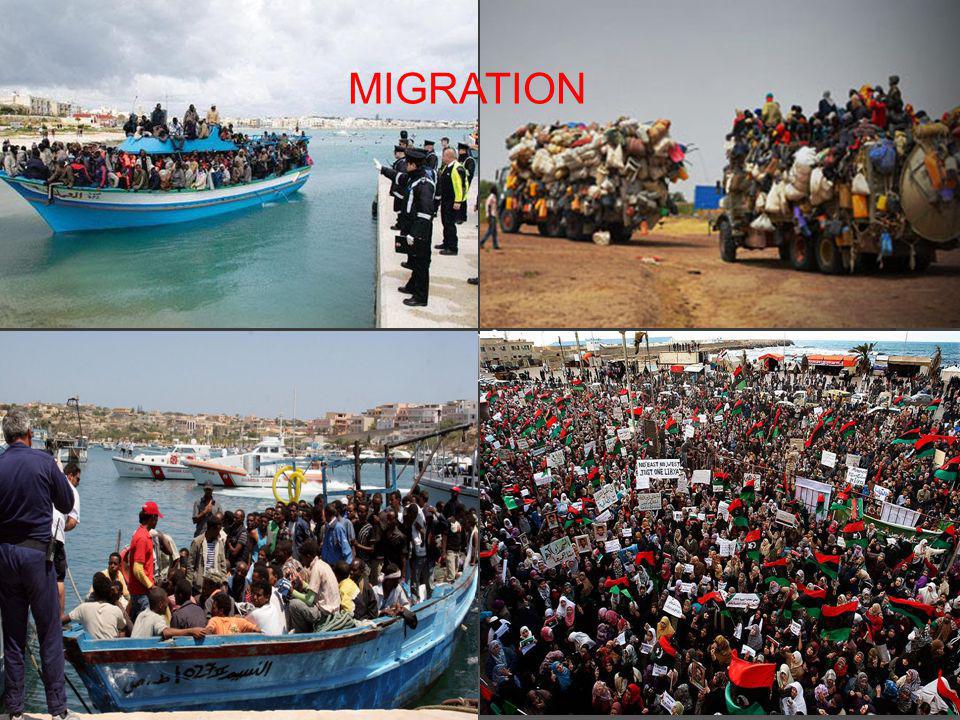This image, titled "Migration" in bold red letters at the top center, is divided into four distinct panels separated by black lines, each depicting various scenes of mass migration. 

In the top left panel, a blue and white boat teeming with possibly thousands of people is nearing a dock. Among the crowd, security personnel in black uniforms with white stripes can be seen. The background features a cloudy sky and a cityscape with buildings and some hotels.

The top right panel illustrates a caravan of two large trucks overloaded with people and their belongings, with bags hanging off the sides. The migrants are densely packed, struggling for space.

The bottom left panel shows another crowded blue boat arriving at a dock, this one containing dozens of people. The scene includes several other boats in the surrounding waters, indicating a busy and possibly chaotic migration event.

In the bottom right panel, a large crowd of people appears to be protesting with signs. The crowd is dense, with a sea of faces and flags visible. The specific connection of this protest to the depicted migration scenes seems to be their shared origin or cause.